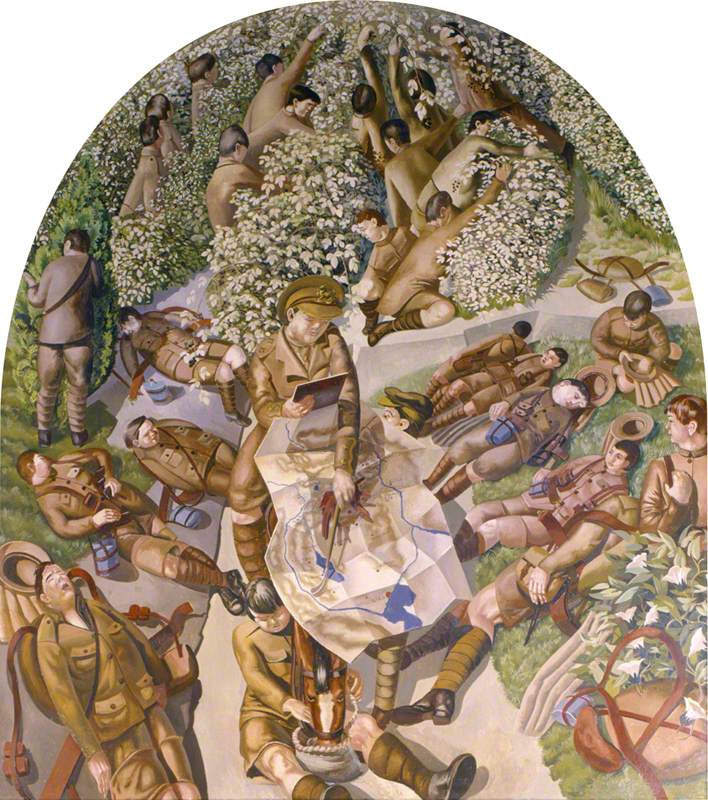This artist's depiction, painted in oils and shaped like a keyhole with a flat bottom and curved top, showcases a detailed garden scene bustling with activity. The scene is divided into distinct areas, each teeming with figures clad in green and tan uniforms reminiscent of army or park ranger attire. 

In the foreground, several soldiers are in various states of rest or sleep, sprawled on a grassy field next to a sidewalk. Their hats are off, and they wear cargo gear, some partially undressed, illustrating their exhaustion. Towards the middle, a prominent figure sits elevated, distinguished by a fancy military cap. He holds a clipboard in his right hand and a large map in his left. Nearby, another soldier tends to him, possibly washing his feet with a bowl of water placed between his legs.

In the background, a different type of activity unfolds. About ten individuals with black or brown hair and light skin are diligently picking white flowers or perhaps cotton from bushes, unconcerned with those resting. These workers wear similar uniforms and shorts, emphasizing their communal task amidst burgeoning white blooms.

This richly detailed scene encapsulates a juxtaposition of labor and rest in a verdant garden, capturing the essence of weary soldiers and industrious workers in harmonious coexistence.